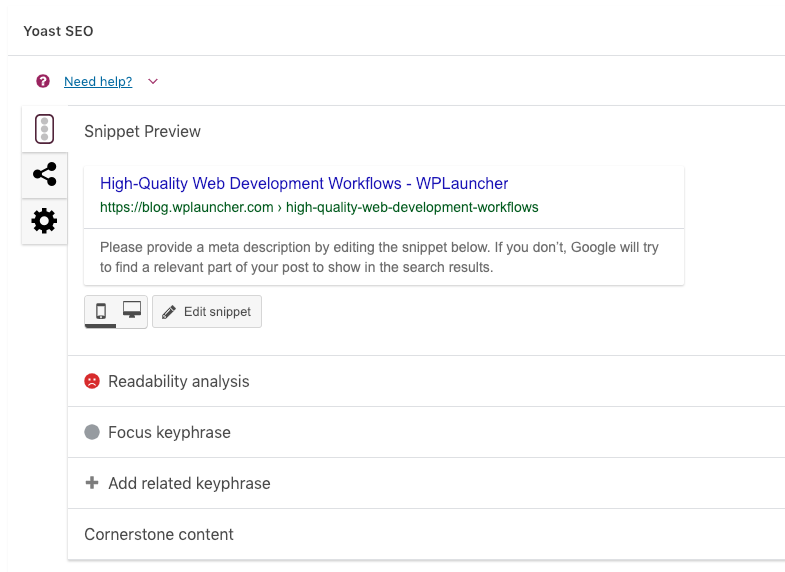The top left corner of the image displays the logo for "Yoast SEO," with "Yoast" spelled Y-O-A-S-T. Directly below, there's a red circle containing a white question mark. Next to it, in blue and underlined text, it says "Need help?" with the question mark. Below this, the section titled "Snippet Review" is followed by a headline in blue that reads "High Quality Web Development Workflows - WP Launcher." 

The URL "https://blog.wplauncher.com" appears below, with an arrow pointing to the right, and the phrase "high-quality-web-development-workflows," each word separated by dashes. Continuing down the image, there is a prompt instructing users to "Please provide a meta description by editing the snippet below. If you don't, Google will try to find a relevant part of your post to show in the search results."

Further down, there are images of a cell phone and a computer, adjacent to the option labeled "Edit Snippet." Underneath, the image shows headings for "Readability Analysis," "Focus Keyphrase," "Add Related Keyphrase," and "Cornerstone Content."